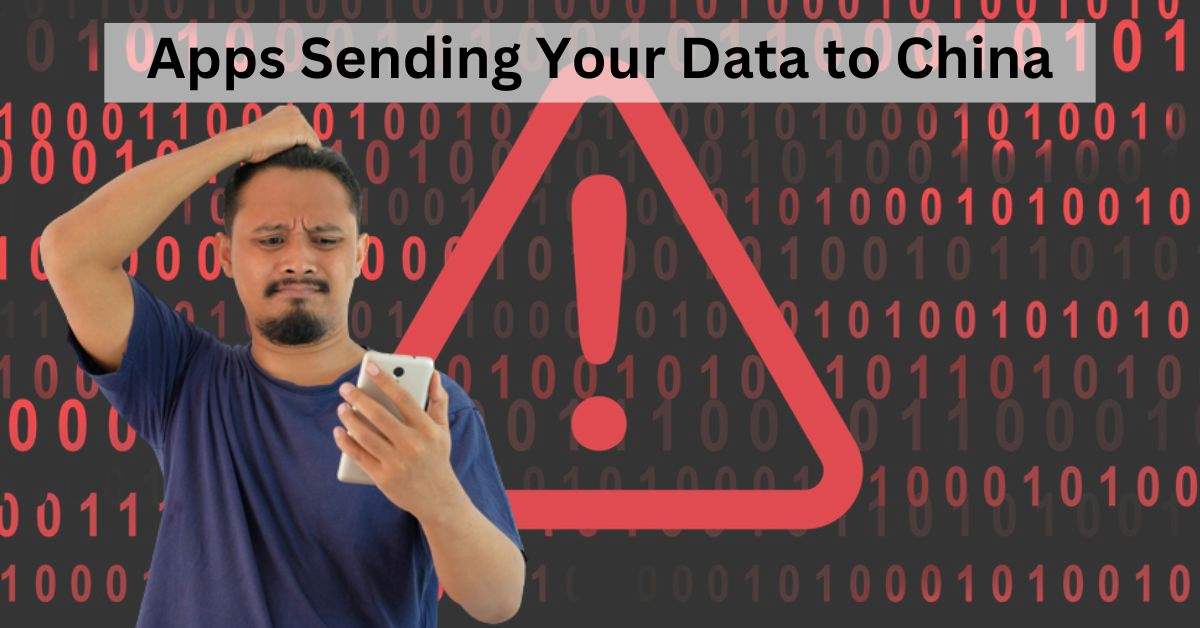The image appears to be an advertisement designed to raise awareness about data privacy concerns. It is a large, horizontal rectangle with a dark grayish-black background, creating a stark and serious tone. Scattered across this backdrop are red numbers, primarily zeros, and ones, evoking a sense of digital complexity and possibly hinting at data streams or binary code.

In the center of the advertisement, a white translucent rectangle provides stark contrast to the dark background, displaying the text, "Apps Sending Your Data to China" in bold black letters. This prominent message captures the viewer's attention immediately.

Dominating the central area is a large red triangle with a red exclamation point inside, outlined vividly to draw focus. This triangle is a classic warning symbol, suggesting a significant issue or alert.

Off to the left of the red triangle stands a man, appearing perplexed and concerned. He has short, dark brown hair, a mustache, and a goatee. He seems to be of Hispanic descent. Dressed in a blue shirt, he holds a white phone in his right hand, which he is staring at intently. His other hand rests on his head, further emphasizing his confused and troubled demeanor. His furrowed eyebrows and overall expression convey his alarm and uncertainty about the information on his phone.

The image effectively combines visual and textual elements to evoke a sense of urgency and concern about data privacy, specifically related to apps potentially sending user data to China.